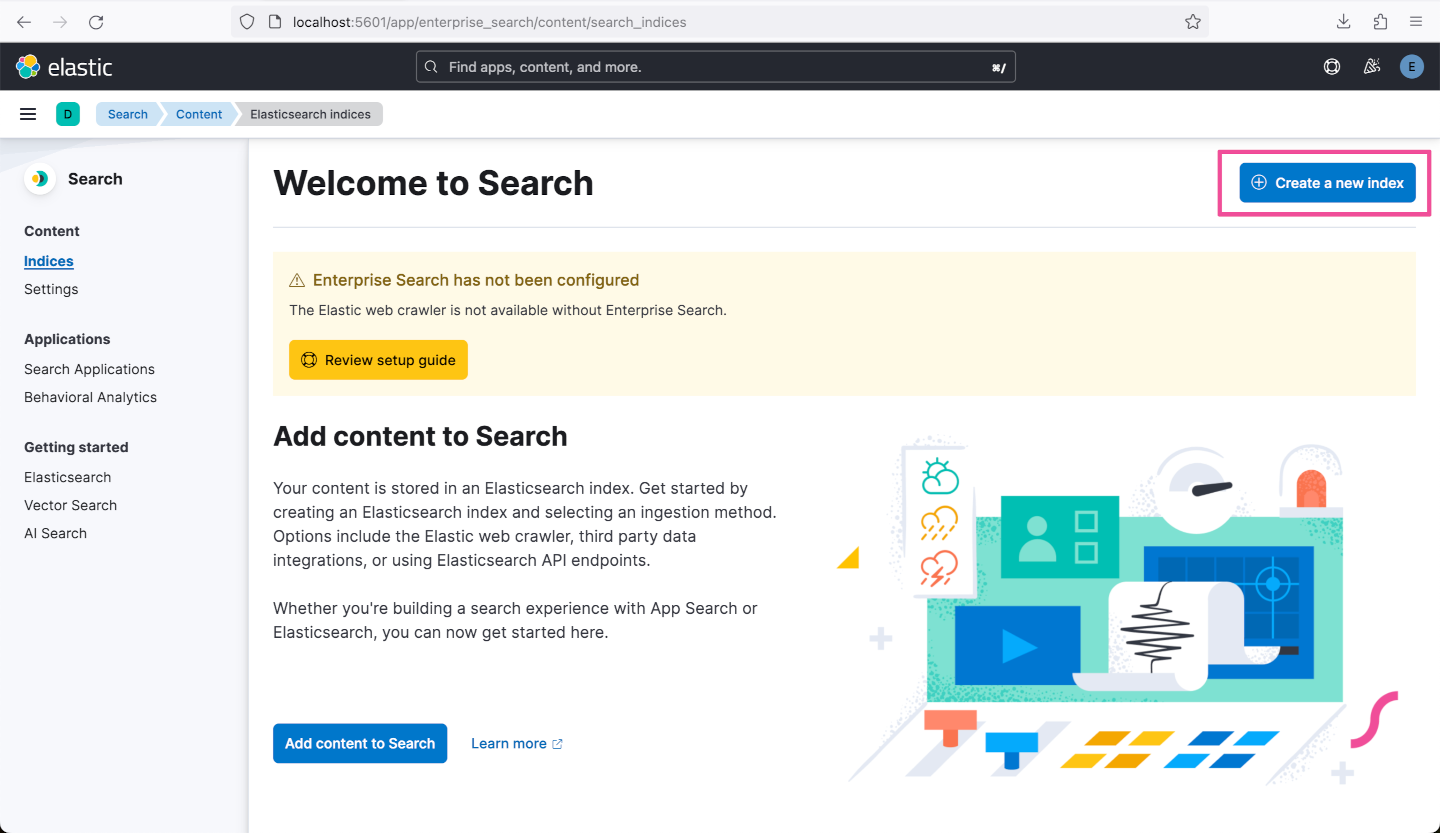The image displays a browser window with the URL "localhost:5601/app" open. The website features a header with a predominantly black background. On the left side of the header, the word "Elastic" is displayed alongside a collection of colored circles in yellow, green, blue, pink, and green. On the right side of the header, there is a search bar labeled "Find apps, content, and more," followed by an icon for user login or profile.

Below the header, a main section displays the text "Search content - Elastic search indices." On the left side of this section, a vertical menu is visible, listing various options such as Search content, Indices, Settings, Application search, Application behavior analytics, Getting started, Elastic search, Vector search, and AI. The "Indices" option is selected and highlighted in blue.

On the right side of the screen, the title "Welcome to Search" is prominently featured. Accompanying this title is a blue button with the label "Create a new index," which is also highlighted with a pink rectangle.

Under the "Welcome to Search" section, there is text indicating that "Enterprise Search has not been configured. The Elastic web crawler is not available without Enterprise Search." An orange button labeled "Review setup guide" follows this text.

Further down, there is instructional text explaining how to add content to search. It mentions that content is stored in an Elasticsearch index and provides steps for beginning the process by creating an index and choosing an ingestion method. Options include the Elastic web crawler, data integrations, or using Elasticsearch API endpoints. The text concludes by encouraging users to get started with search experiences using App Search or Elasticsearch.

At the bottom of this section, two buttons are displayed: a blue button labeled "Add content to search" and another button labeled "Learn more."